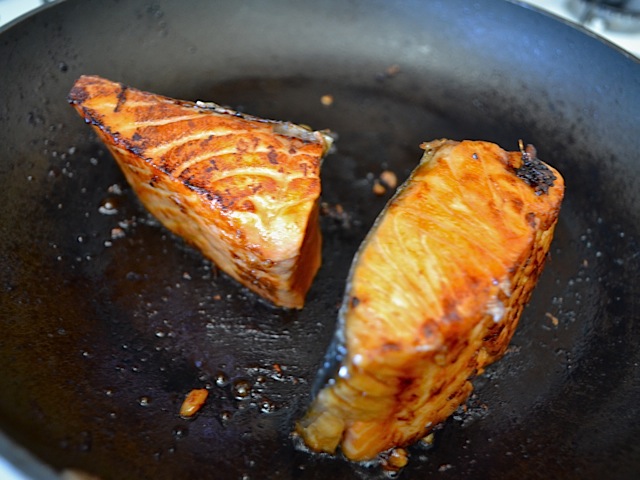The image depicts a close-up view of a black frying pan containing two pieces of salmon fillet. The salmon, a vibrant orange-pink color with white stripes and some dark char marks, is balanced on its cut sides, revealing the fish's grain. The fillets, cooked through and possibly a bit overdone, show signs of browning. The pan's interior is greasy and littered with small chunks of fish and burnt crisps. The salmon pieces are oriented differently: the left fillet, triangular in shape, points to the left and slightly upwards, while the right fillet, more rectangular, points mostly upwards and slightly to the right. The frying pan extends to the edges of the image, cutting off at the borders, and the background in the upper and lower corners is visible but indistinct.